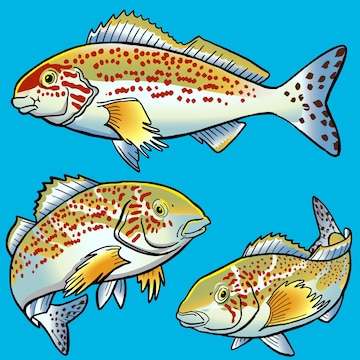The image is a high-quality digital illustration depicting three fish swimming across a bright blue background. The fish appear to resemble either trout or salmon, with distinctive features highlighting their striking coloration. The fish have light green upper bodies that transition into white and light tan undersides. Their bodies are adorned with numerous red polka dots and larger dark blotches, particularly along the sides and tail fins. The fins are detailed with yellow tips, and the dorsal fins on their backs are elongated and white. The fish's tail fins are white with additional red spots. The top fish is shown sideways, displaying the entire length of its dorsal fin extending toward its tail, while the remaining two fish swim beneath it, positioned to show their sides and partially their tails. The illustration captures the dynamic and vividly colorful nature of the fish in a stylized manner against the sky-blue background, devoid of any text or other objects.